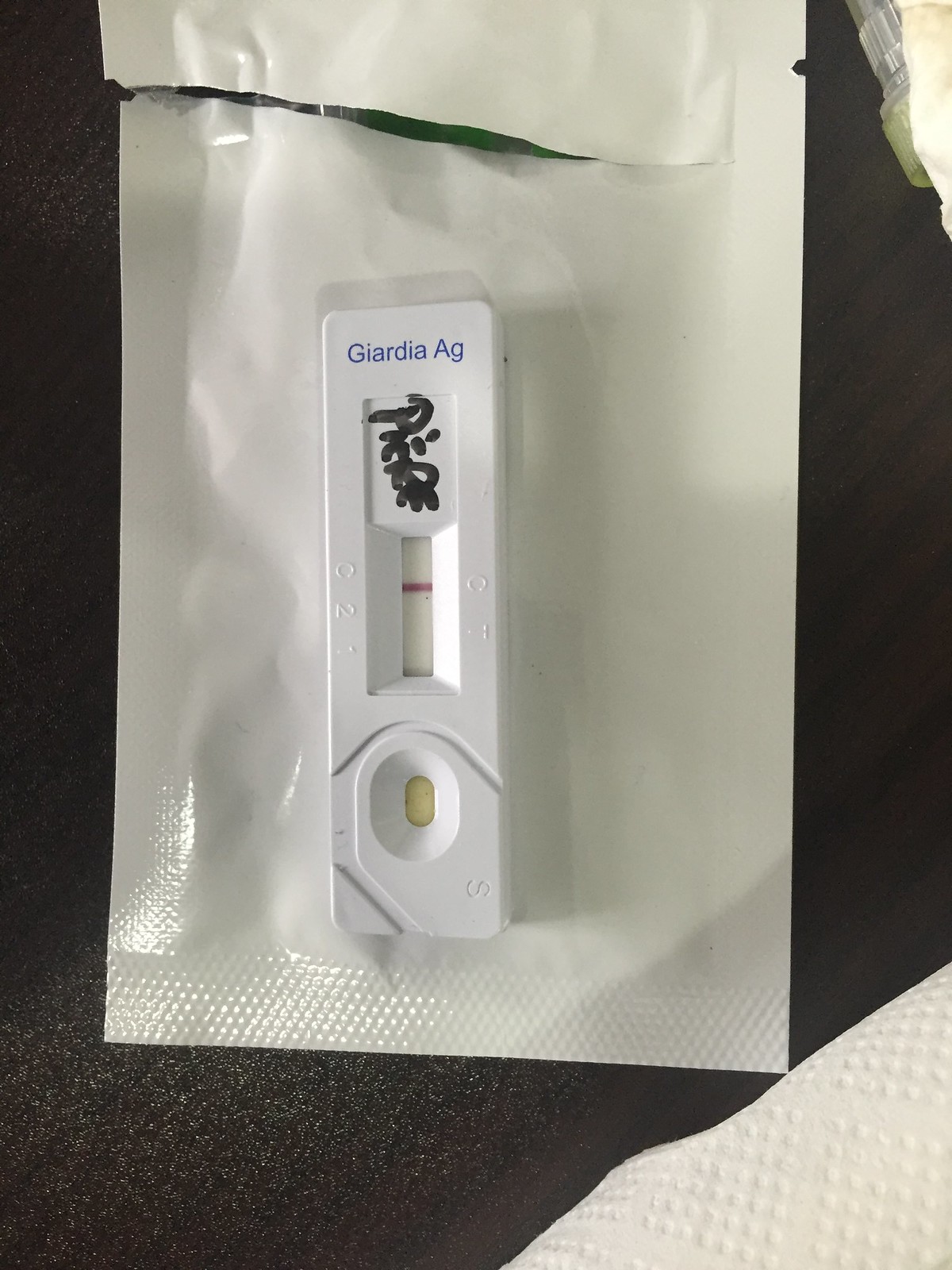The image depicts a partially opened COVID test kit manufactured by Giardia AG. The white test kit remains in its packaging, albeit the packaging has been noticeably broken open. Above the test kit, something illegibly scribbled with a black marker, beginning with the letter "P," is visible. The test kit features two indicators labeled 'C' and 'T.' A distinct red line runs across the 'C' indicator, while the 'T' indicator is blank. These sections are separated by a swirly, indented line. Additionally, the kit includes a clear oval image and a diagonal image on the left-hand side. The brand name "Giardia AG" is printed in blue on the kit. The opened packaging lays atop its original, now opened package, possibly not entirely reinserted. The entire setup rests on a black surface. The lower right corner of the image shows a paper towel, which may be from a roll or a single sheet. In the upper right-hand corner, a round plastic object with a green end is partially overlaid by a white item.